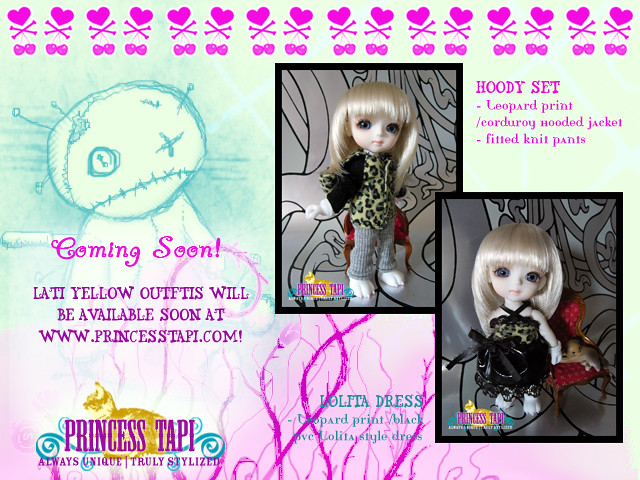This advertisement poster promotes Princess Taupe's upcoming collection of doll clothing, featuring detailed and colorful text and images. On the left side, in purple text, it announces, "Coming Soon: Lati Yellow Outfit will be available soon at www.princesstape.com." Below this, the company name, "Princess Taupe," is displayed with the tagline, "Always Unique, Truly Stylized." The bottom middle section features blue text, highlighting "Lolita Dress Leopard Print," and describes it as a "black Lolita style dress." Adjacent to this is a photo of a doll in a black dress.

Above this section, another doll is showcased wearing a shirt and pants, with the adjacent pink text describing the "Reset Leopard Print / Corduroy Hooded Jacket and Fitted Knit Pants." Notably, both dolls have blonde hair and blue eyes. In the background, a blue and pink patterned stuffed toy can be seen, adding to the visual appeal. At the top, a row of pink hearts decorated with crossbones and cherries contribute to the whimsical and slightly gothic theme. The overall design gives off a playful yet dark vibe, with hues of purple, pink, and black dominating the color scheme, accentuating the unique, stylized nature of Princess Taupe's doll fashion.